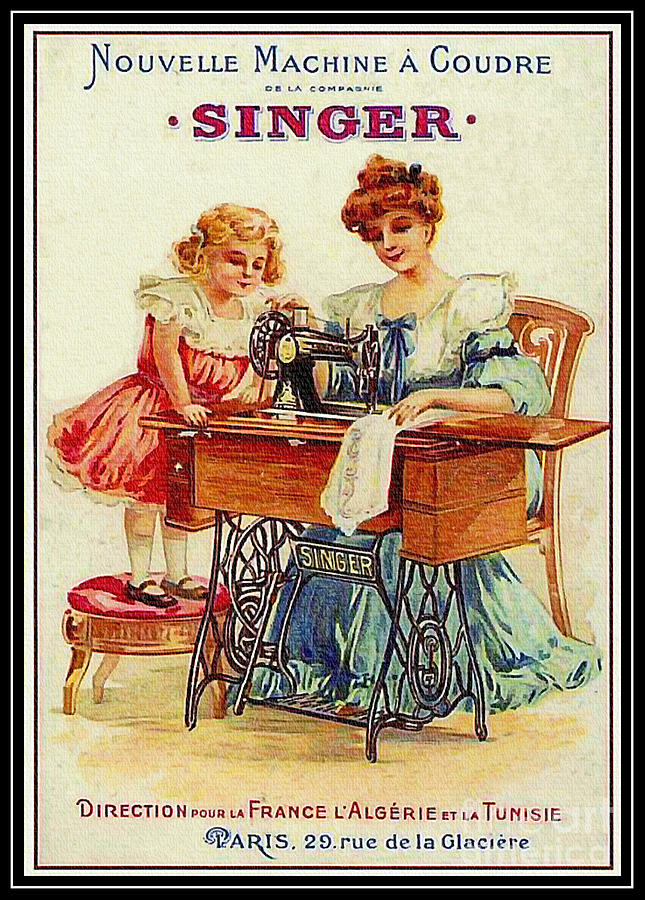This full-page magazine advertisement from the turn of the 20th century showcases a classic Singer sewing machine in a beautiful, vintage illustration. Enclosed within a narrow black frame, the background of the advertisement features aged, textured paper. The top of the ad is adorned with French writing in blue that reads "Nouvelle Machine à Coudre," followed by "Singer" in red. In the center of the illustration, a woman with her hair elegantly pinned up with blue ribbons sits on a wooden chair. She is engaged in sewing a piece of white cloth using a pedal-operated Singer sewing machine, which is built into a wooden cabinet with an iron undercarriage emblazoned with the brand name "Singer." Her right hand skillfully operates the large wheel while her left guides the fabric under the needle. To her left, a young blonde girl with her hair tied in pigtails with white ribbons stands attentively on a red, three-legged stool. She is wearing a red dress with lace trim around the collar and shoulders and black Mary Jane shoes. The bottom of the advertisement also contains additional French text, completing this vintage promotional piece with an air of timeless elegance.